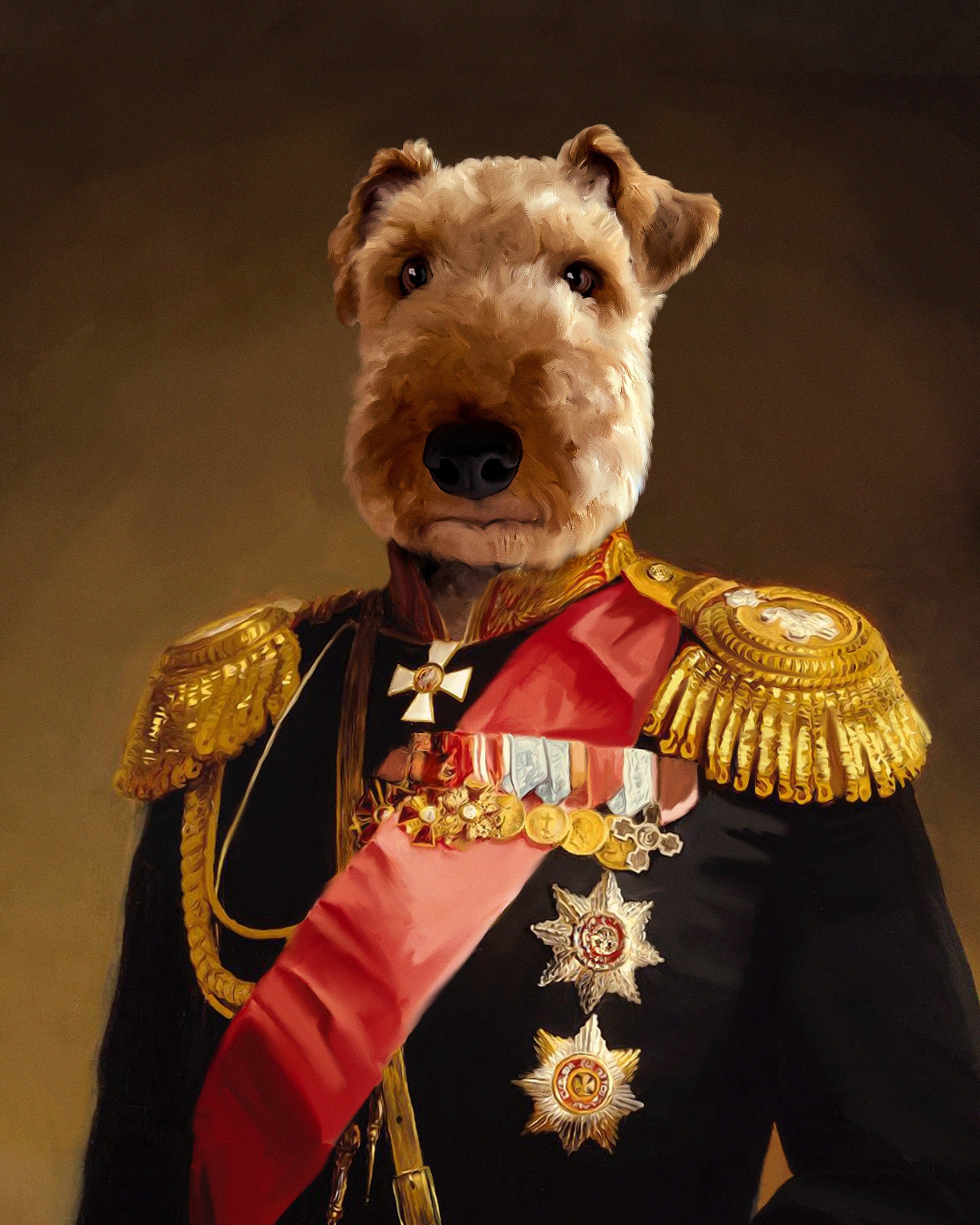This detailed and richly decorated painting features a terrier-type dog standing upright, dressed in an elaborate military uniform. The uniform is primarily black with intricate gold detailing, including shoulder pads adorned with golden tassels, known as epaulets. A striking red sash runs diagonally from the right shoulder to the left waist, accentuated by a row of medals pinned across it. The left side of the chest boasts two large star-shaped medals, each with numerous points, while gold chains elegantly drape from the left shoulder beneath the sash. A prominent Maltese cross is visible at the center of the uniform. The dog's fur is a golden-blonde color, with a very fuzzy face, floppy ears, and a black nose, conveying a mix of noble stature and endearing charm. The background of the portrait transitions from dark chocolate brown at the top to lighter honey brown and olive hues towards the bottom, providing a classic and dignified setting for the distinguished canine subject.